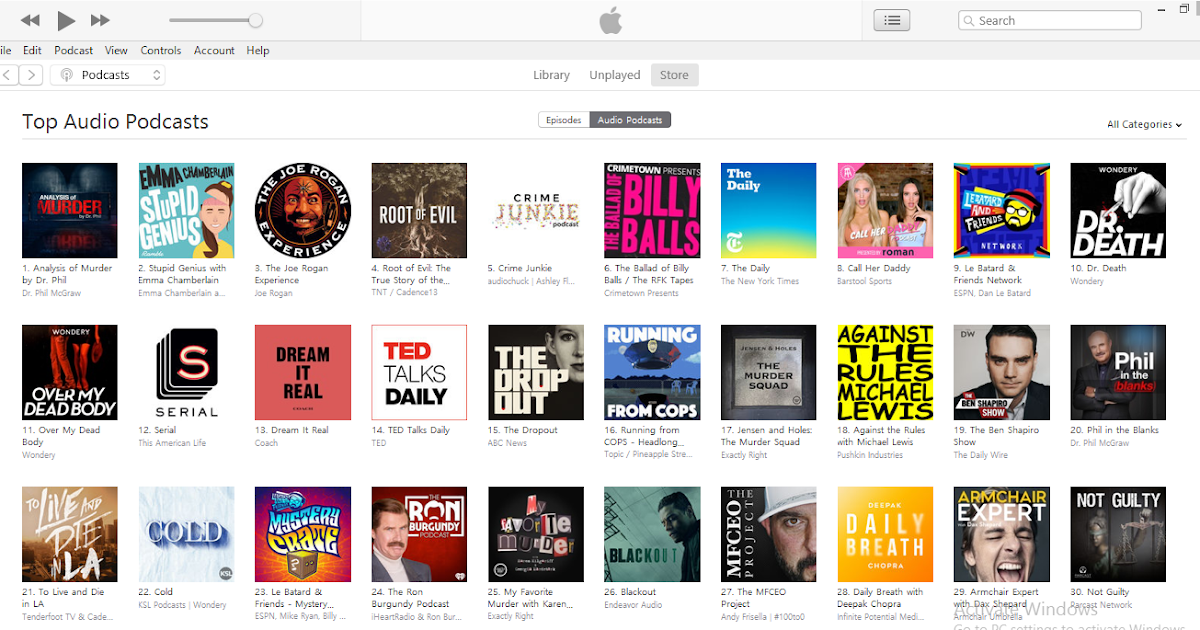The image displays a vibrant and colorful webpage featuring various podcasts on an Apple computer. At the top of the page, prominently centered, is the Apple logo adjacent to a search bar, making it convenient for users to search for specific podcasts. The header prominently displays the word "Podcasts," instantly indicating the theme of the webpage. Below, the text "Top Audio Podcasts" is showcased, surrounded by a diverse array of podcast thumbnails featuring faces, logos, and intriguing graphics. Among them, notable podcasts include one titled "Root of Evil" with a tree graphic, and another named "Stupid Genius," illustrating the wide variety of content available.

The search bar allows users to input their preferences, with options to categorize search results via a dropdown arrow labeled "All Categories." Additional navigation options include "Auto Podcasts" and "Episodes," presented in a sleek black and white format. Beneath the Apple logo, there are tabs for "Library," "Unplayed," and "Store," providing multiple pathways to explore, organize, and select podcasts according to personal interests. On the upper left-hand corner of the screen, a large arrow button is visible, inviting users to play the selected podcast. The vibrant interface and user-friendly navigation underscore the platform's extensive podcast offerings.